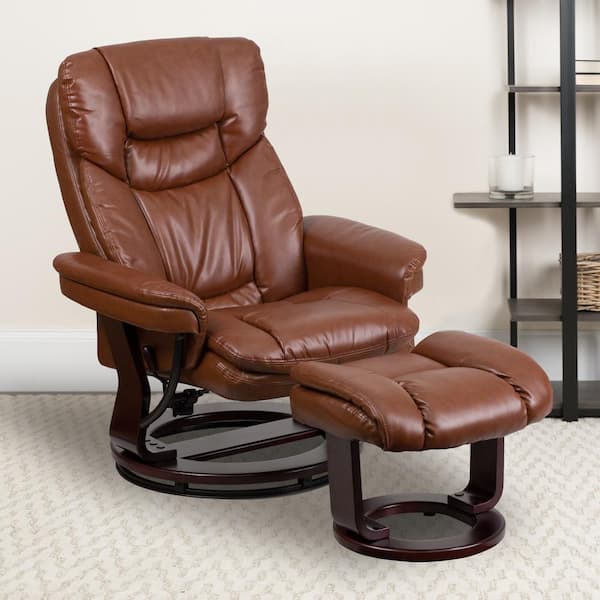This indoor color photograph features a brown leather reclining easy chair with a matching leg rest ottoman. The chair, with its high headrest and padded armrests, and the ottoman both have circular, dark brown wooden bases. The leather appears to be lighter in shade compared to the wood. The chair and ottoman are situated on a zigzag or chevron-patterned wall-to-wall carpet. To the right, there's a black bookcase with four visible shelves. Various decorative items, including a wicker basket on the second shelf and a glass vase containing a white candle on the third shelf, adorn the bookcase. Behind the chair and bookcase is a plain white wall.